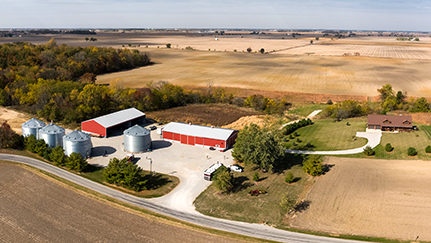This aerial daytime photograph captures a sprawling farm with extensive tan and yellow fields that may be used for wheat or corn cultivation. The expansive landscape is punctuated by large machinery, including substantial tractors. Highlighted prominently in the midline of the image are two large red metal barns accompanied by four shorter gray metal silos. To the right of these agricultural structures, a road leads to the family home, situated about 500 feet away, and features a well-kept lawn and a circular driveway. This single-story tan house with a brown tile roof is framed by trees in the background. The skyline is a pale blue with a hint of gray haze, contributing to the serene rural setting of this compact but detailed image.